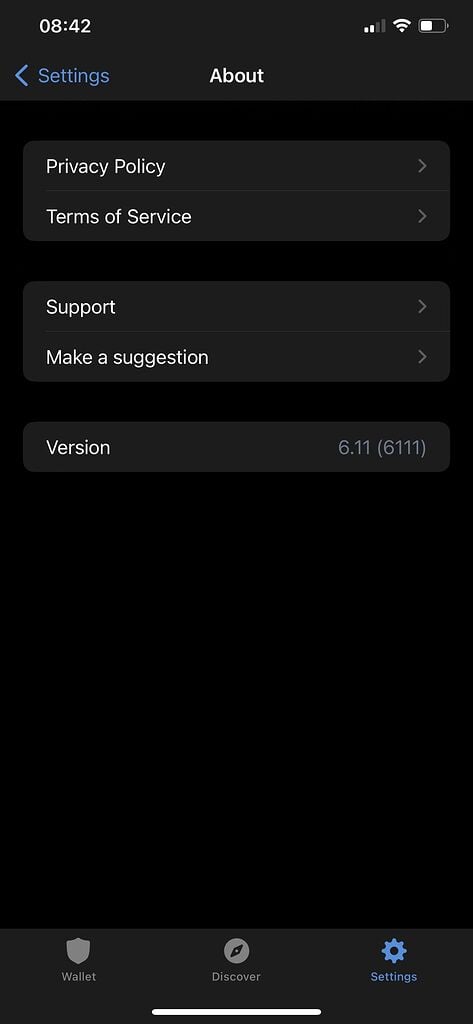The image depicts a cell phone screen with a predominantly black background, featuring various interface elements. At the top left corner of the screen, the time is displayed as "08:42" in white letters. On the top right, there are indicators showing a "2 out of 4 bars" signal strength and a battery icon that is about half full.

Directly below the top bar, the background changes to a dark gray. This section includes a blue left-facing caret and the word "Settings" on the left, and the word "About" in white in the center.

Following this, the screen returns to a black background with two options displayed on gray backgrounds. The first option is "Privacy Policy" in white letters with a right-facing gray caret at the far right. The second option, also on a gray background, is "Terms of Service" in white, accompanied by another right-facing gray caret.

Below these options, the screen remains black until two more menu items on gray backgrounds are visible. The first is labeled "Support" and the second "Make a Suggestion," both in white letters and each with a right-facing gray caret.

Beneath these options, the screen stays black until the last option appears on a dark gray background. This final option reads "Version" in white letters, and to its far right, it displays "6.11 (6111)" in gray letters.

The bottom half of the screen remains black except for a dark gray band at the very bottom, which contains three icons: "Wallet," "Discover," and "Settings." The "Wallet" and "Discover" icons are gray, while the "Settings" icon is highlighted in blue.